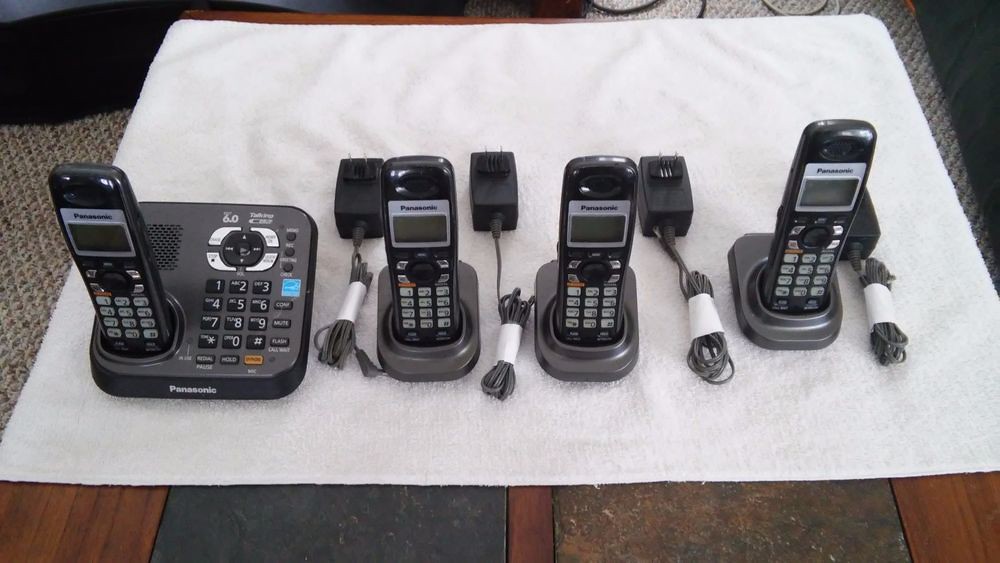This detailed photograph captures a set of four Panasonic cordless landline phones arranged on a piece of white terrycloth, which is placed over a wooden table with a stone inset. The scene appears to be indoors, likely prepared for listing items online for sale. 

On the far left is the main handset in its base, which features a wide base equipped with a speaker, number keypad, and voicemail buttons. The phone is upright and appears to be in excellent or like-new condition. The three additional handsets are positioned in a row to the right of the main unit, each nestled upright in smaller, simpler charging bases devoid of keypads. Next to each base are neatly bundled power cables and chargers, securely taped together for organization. Overall, the setup suggests that this is a comprehensive home phone system designed to allow handsets to be placed and used in multiple rooms within a house.